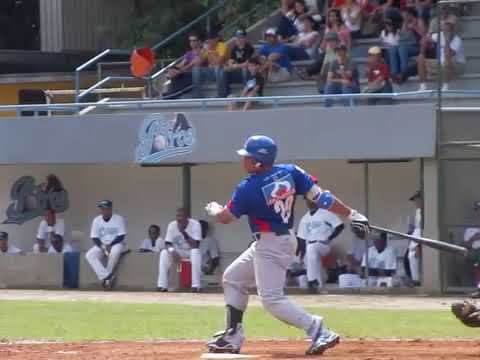In this image of a baseball game, the primary focus is on a player with darker skin, who has just completed a swing. The player is wearing a blue jersey with the number 20 on it, a blue helmet featuring a white Adidas logo, blue elbow guards, and white batting gloves. His pants are white, and he has on black and white shoes. The bat, black in color, is held in his right hand, extended straight back behind him, while his left arm is bent across his chest. He appears to be poised, almost ready to run. 

In the background, there are two layers of people. The bottom layer comprises dark-skinned players of the opposing team who are wearing white jerseys, white pants, and black hats; some of them are bald. They are situated in the dugout, above which a protective covering is present. There is some indecipherable light blue text and possibly a baseball icon above them, suggesting it might be a high school stadium since the setting appears less professional. Above the dugout, the audience is seated on long metal benches, dressed in casual attire, attentively watching the game.